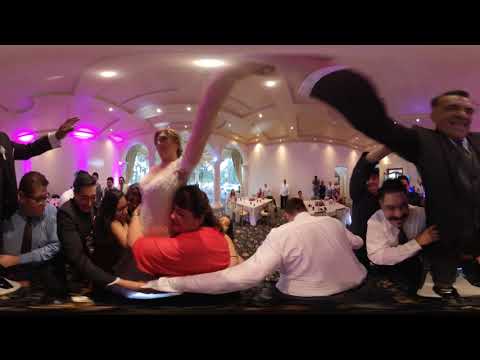This indoor photograph, likely captured at a celebration or party, presents a distorted image with black bars at the top and bottom, possibly indicating it is a screenshot from a video. The setting features a flowered carpet and tables dressed with white tablecloths, suggesting a formal event in a reception hall. The central scene includes various people engaged in hugging and dancing. A Caucasian woman, potentially a bride in a wedding dress, is on the left with her left arm raised dramatically. She is being embraced from behind by a woman with brown hair in a red dress. On the right, a man with brown skin in a black suit and tie appears to be holding the bride's hand while another man stands behind him, holding onto his waist. Their exaggerated gestures and body proportions are humorously distorted due to a bubble effect, making their arms appear disproportionately large and their bodies shrunken. This effect also comically distorts a man's head, magnifying his body in comparison. The background features more guests, some seated and some standing, adding to the lively and chaotic ambiance of the celebration.